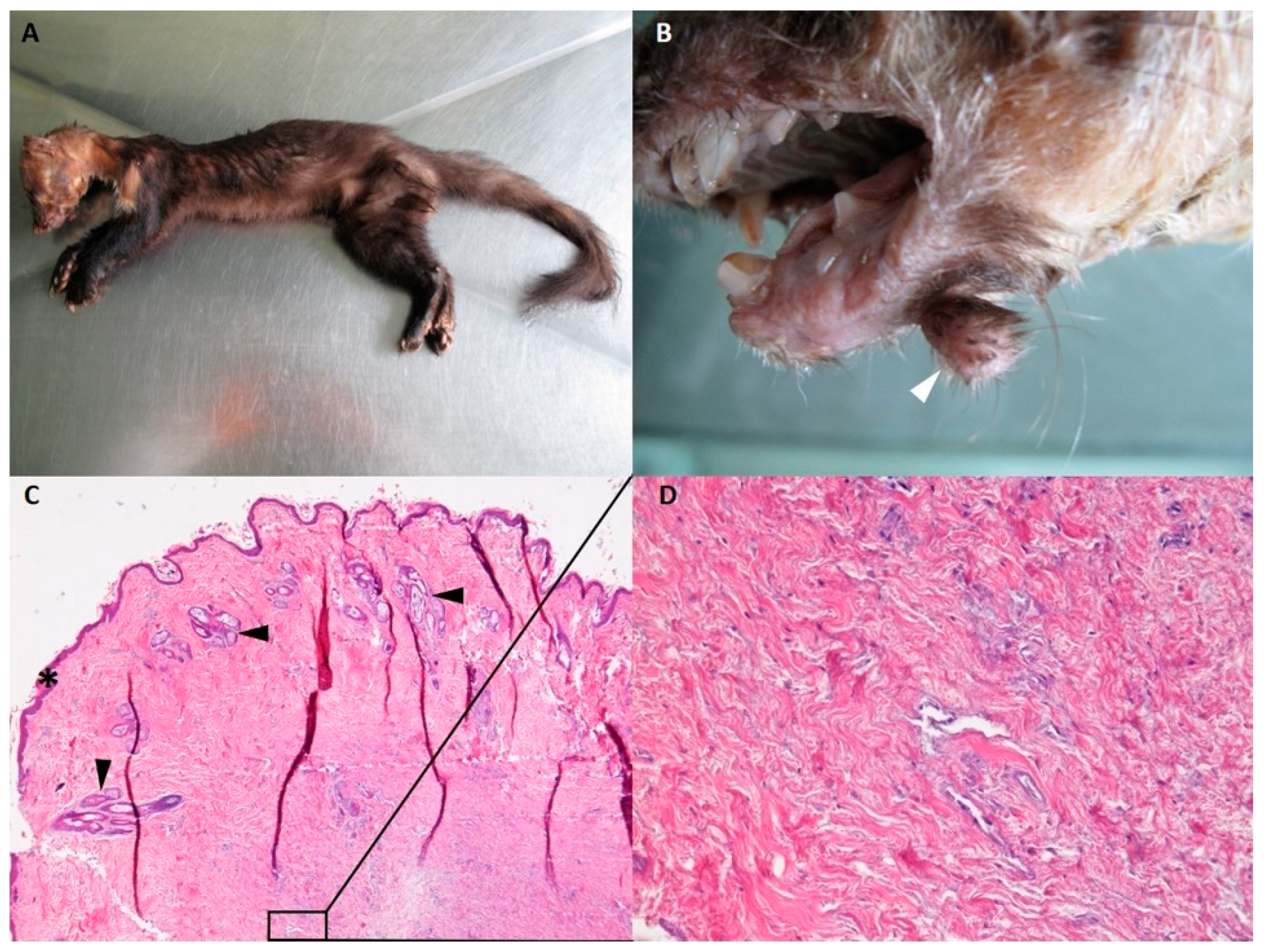The image depicts a deceased cat, likely subjected to a pathology examination, composed of four distinct frames labeled A, B, C, and D. 

**A**: In the top left, the emaciated and severely deteriorated cat, lying on a steel table, displays significant hair loss, primarily black to brown-hued fur sparse on its sides and back. The ribcage is prominently visible, indicating extreme weight loss. 
**B**: The top right panel offers an inverted close-up view of the cat's mouth, emphasizing a lesion or tumor beneath the jawbone, marked by an arrow. 
**C**: The bottom left frame showcases a microscopic scan with black arrows indicating a possible biopsy of the lesion, presenting in pink, purple, and white hues.
**D**: The bottom right is a magnified section of C, highlighted by a black box in C with an arrow pointing towards D, detailing cellular structures possibly linked to a clinical diagnosis of disease or degeneration. 

Overall, the series of images meticulously document the condition and pathology of the deceased cat with multiple zoom levels to highlight specific areas of clinical interest.